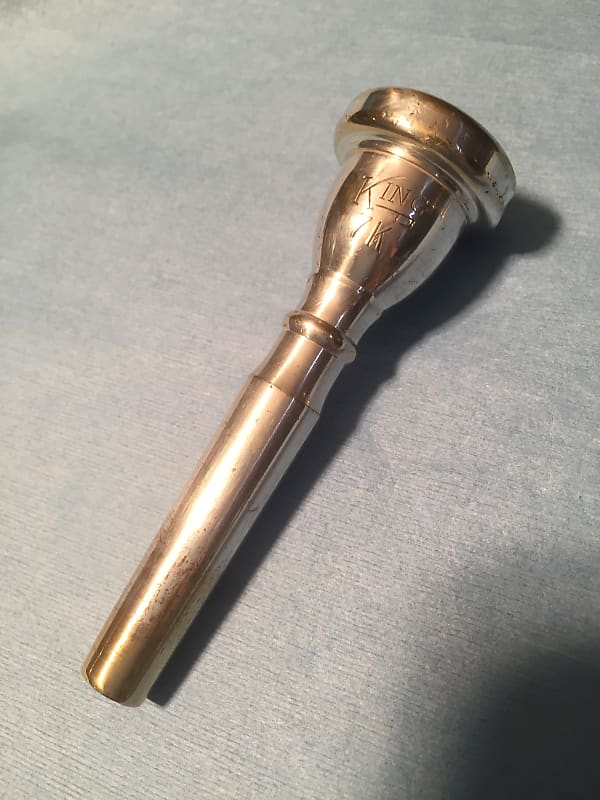The photograph features a close-up of a brass mouthpiece, likely from a trombone or trumpet, placed diagonally against a light blue cloth background with visible shadows. The mouthpiece exhibits a shiny, golden-brass color but shows signs of wear and discoloration, particularly around the area that slides into the instrument. Near the top of the mouthpiece, the engraving reads "King 7K," indicating the brand and model. The mouthpiece has a distinctive long, tube-like structure that widens into a circular bell-shaped end. This well-used piece could be considered an antique relic, displaying pock marks and small damages that suggest its extensive use. The photograph's close-up nature emphasizes the detailed texture and condition of the mouthpiece.